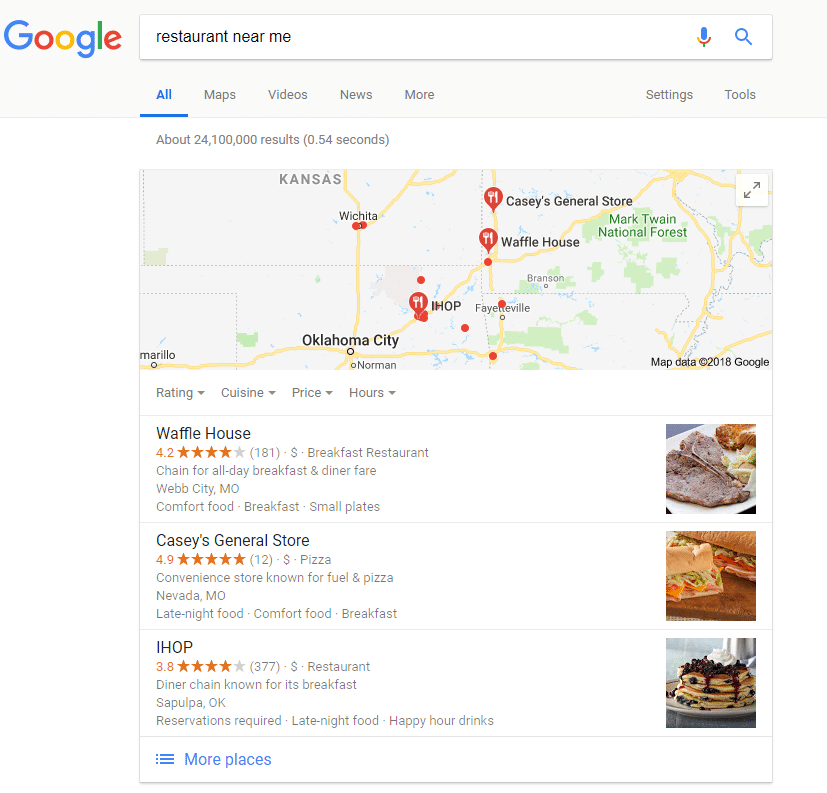Screenshot Description: 

The screenshot showcases a search query on Google.com for "restaurant near me." The search results display a Google Maps section on the right-hand side, highlighting various restaurant locations marked with red dots and small red circles featuring a white fork and knife symbol. Underneath the map, detailed listings of the restaurants are provided. 

1. **Waffle House**:
   - **Description:** Breakfast restaurant chain offering all-day breakfast and diner fare.
   - **Rating:** Not specified.
   - **Price:** Not specified.
   - **Location:** Webb City, Missouri.
   - **Attributes:** Known for comfort food, breakfast items, and small plates.

2. **Casey's General Store**:
   - **Description:** Convenience store renowned for its fuel services and pizza.
   - **Rating:** 4.9 (12 reviews).
   - **Price:** $
   - **Location:** Nevada, Missouri.
   - **Attributes:** Offers late-night food, comfort food, and breakfast items.

3. **IHOP**:
   - **Description:** Restaurant diner chain famous for its breakfast offerings.
   - **Rating:** 3.8 (377 reviews).
   - **Price:** $
   - **Location:** Sapulpa, Oklahoma.
   - **Attributes:** Requires reservations, offers late-night food, and has happy hour drinks.

Each listing provides a concise summary of the restaurant’s key qualities, including its type, rating, price range, location, and notable attributes or offerings.